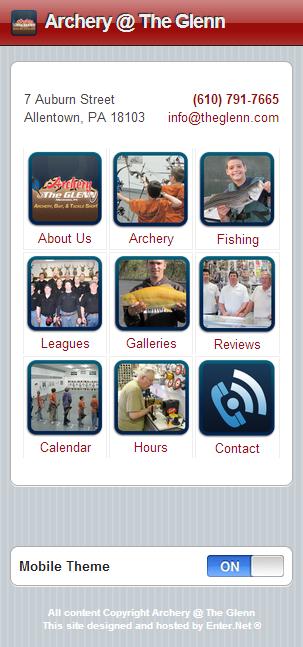The image, set against a vibrant red background, prominently features the title "Archery at the Glen" in bold white letters at the top. Accompanying this title is a black, red, and white symbol. Below the title, the address "7 Auburn Street, Allentown, PA 18103" is printed in black, alongside the contact details in red: "610-791-7665" and "info@theglen.com." The central section of the image is organized into nine sections with small photos and corresponding text labels: "About Us," featuring a child's picture; "Archery," with an image of children in orange attire; "Fishing," showing a kid holding a fish; "Leagues," illustrating a group in black shirts and blue jeans; "Galleons," paired with another child holding a fish; "Reviews," highlighting three individuals in white shirts; "Calendar," depicting a line of children in a gymnasium; "Hours," with someone in a green shirt; and "Contact," symbolized by a phone icon. At the bottom, within a grayish area and white space, an indicator reads "Mobile Theme On" with additional unreadable white text. The overall layout appears to resemble a mobile phone format, enhancing its modern aesthetic.